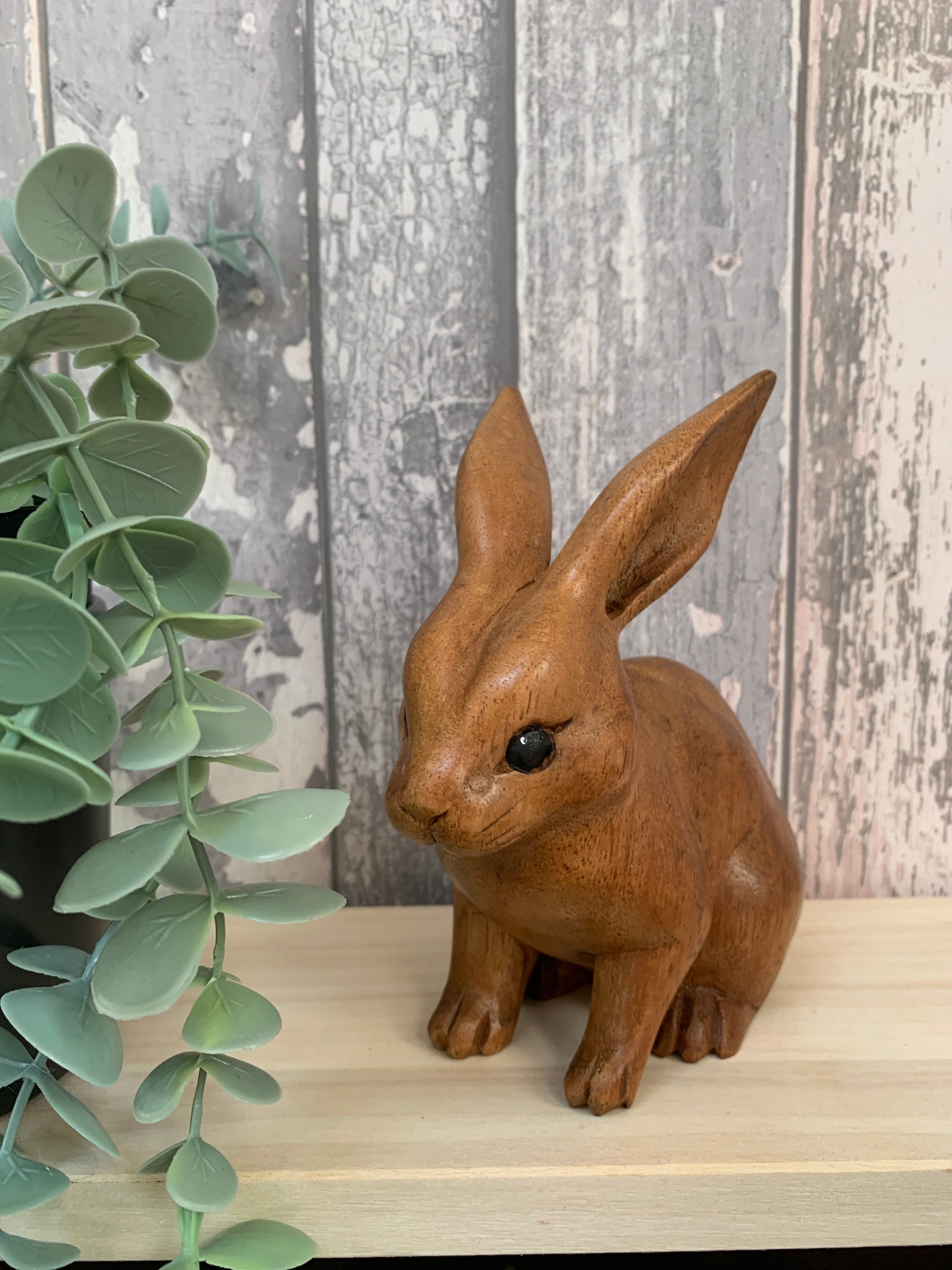The image showcases a highly detailed and realistic wooden carving of a rabbit, finished in a woodish brown color with a smooth, shiny surface, possibly due to sanding and a poly or wax finish. The rabbit is depicted in an alert sitting position, with its slightly back ears revealing carved gullies, a clearly defined nose, and simple notches to indicate toes. A small, beady glass or marble eye is inset, capturing a lifelike appearance. This charming bunny, approximately six to eight inches tall, is positioned on an unfinished light wooden slab. Adjacent to the rabbit is a fake succulent plant, characterized by its green plastic leaves and downward-extending stems. Both items rest against a backdrop of gray weathered wood with beige undertones, giving the scene an outdoorsy feel. The detailed textures and contrasting materials of the rabbit, plant, and background create a visually engaging composition.